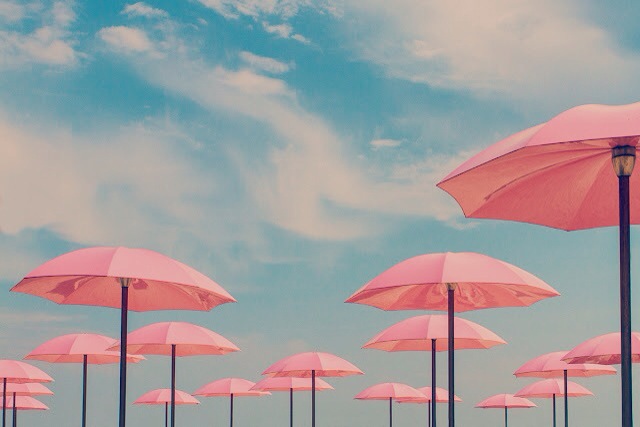This image captures a vibrant, sunlit day under a bright, light blue sky, scattered with delicate, wispy white clouds that resemble stretched cotton candy. Beneath this idyllic sky, rows of large, pastel pink umbrellas are mounted on tall, sturdy black poles. These umbrellas, some displaying varying shades of pink from light to dark, are uniformly spaced, creating an impression of an endless sea of pink. Each umbrella is equipped with a light fixture attached just under the canopy, hinting at their possible permanence and multi-functional use. The overall atmosphere of the image evokes a retro, 80s sunny day vibe, with a touch of graininess enhancing its nostalgic appeal. Though no beach, sand, or water is visible, the scene strongly suggests a picturesque, leisurely environment likely designed for relaxation and outdoor enjoyment.